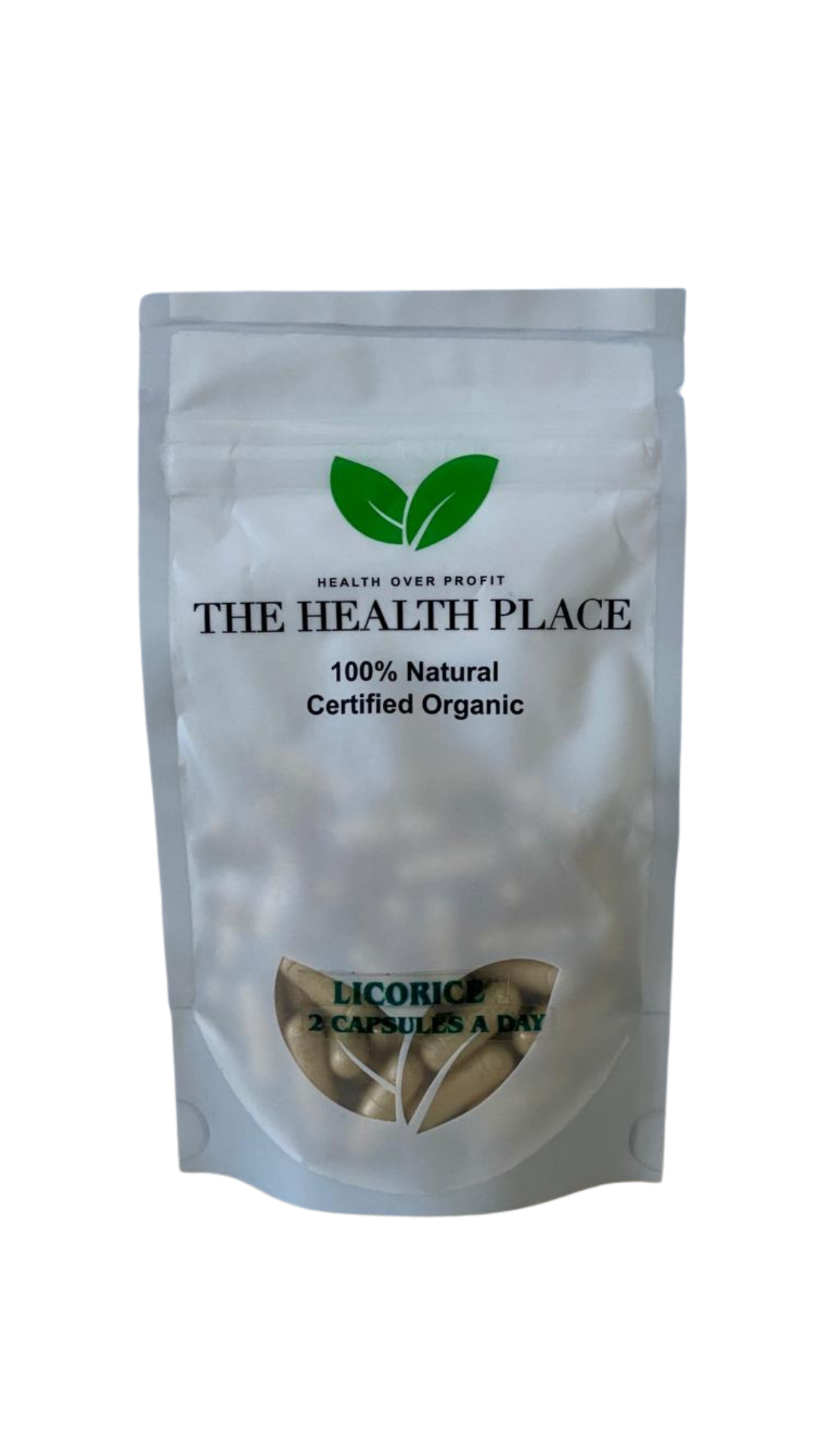The image showcases a plain, flat white package for licorice capsules, offered by the brand The Health Place. The front of the package features a see-through window in the shape of two leaves, allowing visibility of the light brown, cylinder-shaped licorice capsules inside. Above this window, two green leaves are depicted, consistent with the brand's logo. Prominently displayed in bold lettering are the phrases "Health Over Profit" and "The Health Place." Additional text indicates that the product is "100% Natural Certified Organic," with usage instructions recommending two capsules a day.